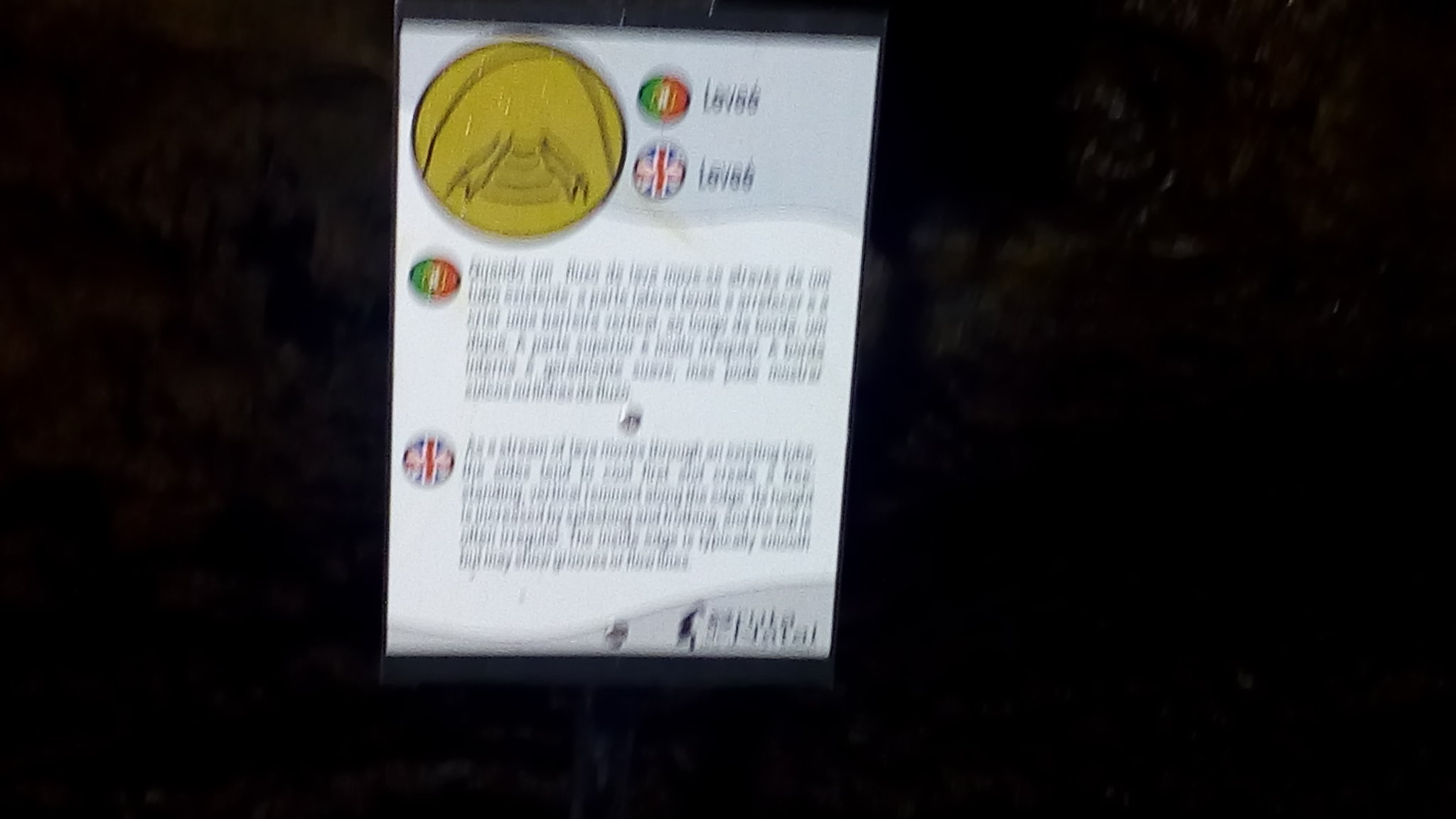A miniature leaflet, its text blurred and difficult to decipher, features several intriguing symbols. On the right-hand side, two circular flag emblems are prominently displayed. The top emblem displays the Union Jack, the national flag of the United Kingdom, while the lower emblem showcases a round representation of the Italian flag, with its distinctive green, white, and red tricolor. The leaflet's left-hand side is adorned with a gold medallion, also in a circular design, positioned adjacent to the flag symbols.

The text beneath the Italian flag appears to be in a different language, suggesting a description or message in Italian. Similarly, the text under the British flag appears to be in English, though the blurriness obscures the exact wording. The purpose of combining the British and Italian symbols on this small leaflet remains unclear.